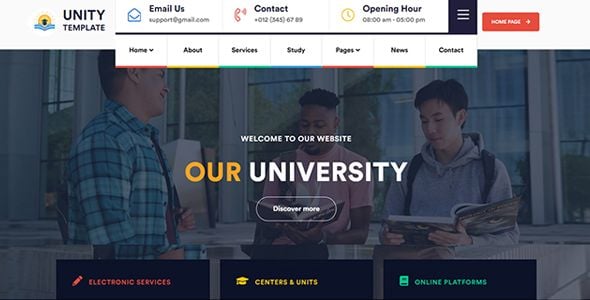This is an image for a Unity Template website featuring educational content. At the top left corner, there's a logo depicting a yellow sun with waves underneath, symbolizing growth and new beginnings. A white banner stretches across the top with navigation options: "Email Us," "Contact," and "Opening Hour." Just below the banner is a black line, underneath which the main navigation menu is displayed. The menu items include "Home," "About," "Services," "Study," "Pages," "News," and "Contact," each highlighted by distinct colors: red for Home, yellow for About, green for Services, blue for Study, red for Pages, yellow for News, and green for Contact.

In the upper right corner, there's a link directing users to the homepage. Beneath the navigation menu, a prominent image showcases three men engaged in a discussion, possibly about their studies, with books in their hands. 

The header text on the image reads, "Welcome to our website, R University OUR," followed by a call-to-action button labeled "Discover More." Below this header, three service categories are listed: "Electronic Services" in red, "Centers and Units" in yellow, and "Online Platforms" in green.

In the foreground, the man on the left wears a blue plaid long-sleeve shirt and is smiling slightly as he looks at his companions, who seem engrossed in their textbooks, likely deliberating on academic topics. The overall scene conveys a warm and collaborative learning environment.